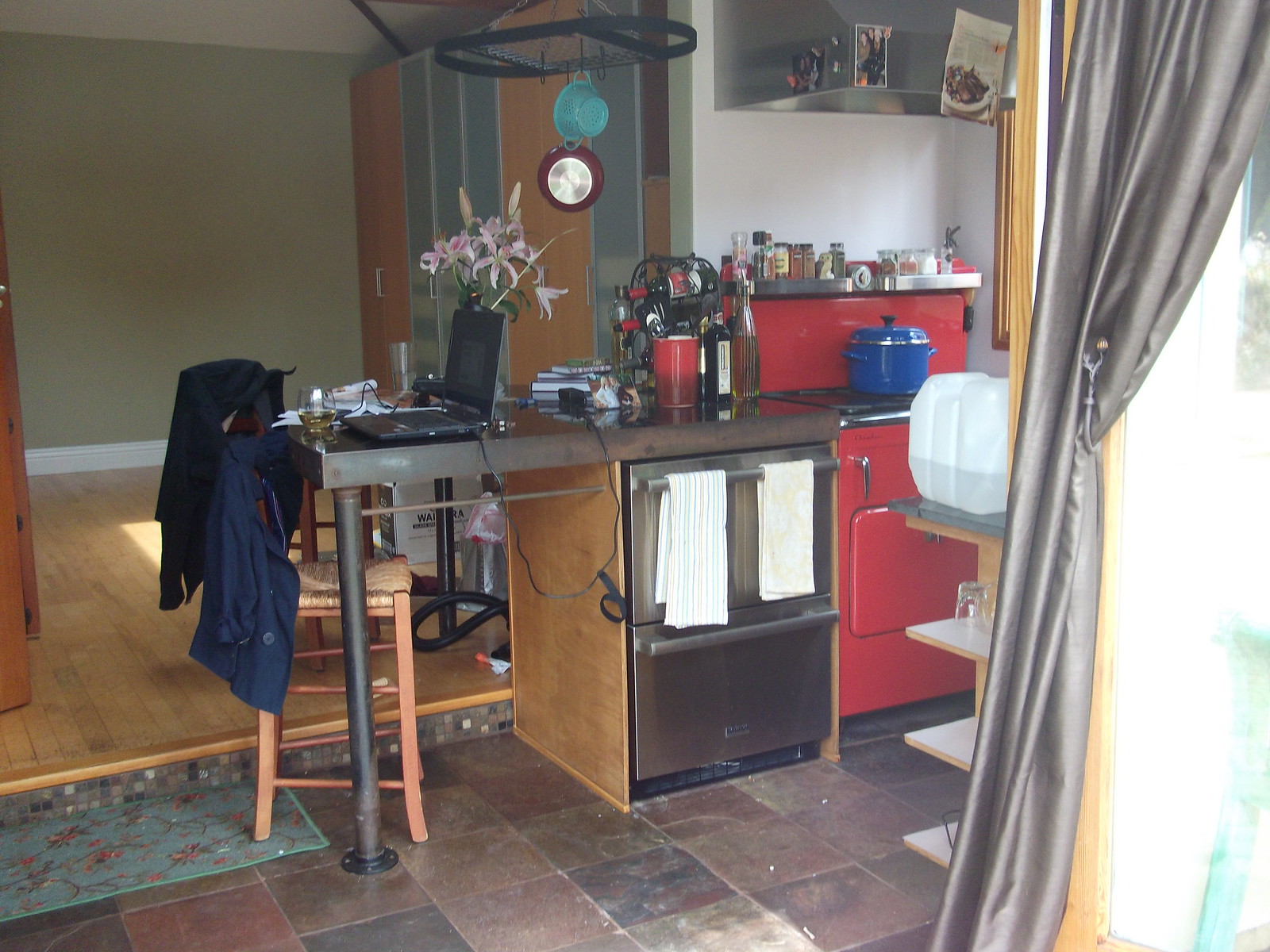This photograph captures a cozy, compact kitchen with a warm, inviting ambiance. The kitchen opens directly into an adjacent room through an opening devoid of a wall but framed by brown doors that seem capable of closing the space off. The floor is adorned with large, brown tiles in a variety of shades—ranging from a rich reddish-brown to darker and even black tones, creating a rustic patchwork effect.

Central to the scene are two stoves positioned side by side. One is a sleek, modern oven with a stainless steel door, while the other is a charming vintage cherry red stove, featuring a red front, red oven door, and matching red backsplash. Atop this stove, a royal blue stock pot with a matching lid sits on a black burner, adding a splash of color to the setting. Adjacent to the red stove, another oven with a steel door displays two white kitchen towels hanging neatly from its handle.

Above the red stove, a stainless steel shelf brims with an array of spices and culinary essentials, adding both functionality and character. The ceiling hosts hanging hooks that hold a skillet and another pot, making efficient use of the limited space. A metal counter, bolted securely to the floor, accommodates a vase of fresh flowers, contributing a touch of nature to the industrial aesthetic.

Beyond the kitchen, the adjoining room stands empty, featuring a light wood floor that contrasts sharply with the kitchen's darker tiles. An olive green wall with a crisp white baseboard forms the backdrop of this vacant space, highlighting the kitchen's bustling charm against the serene simplicity of the next room.